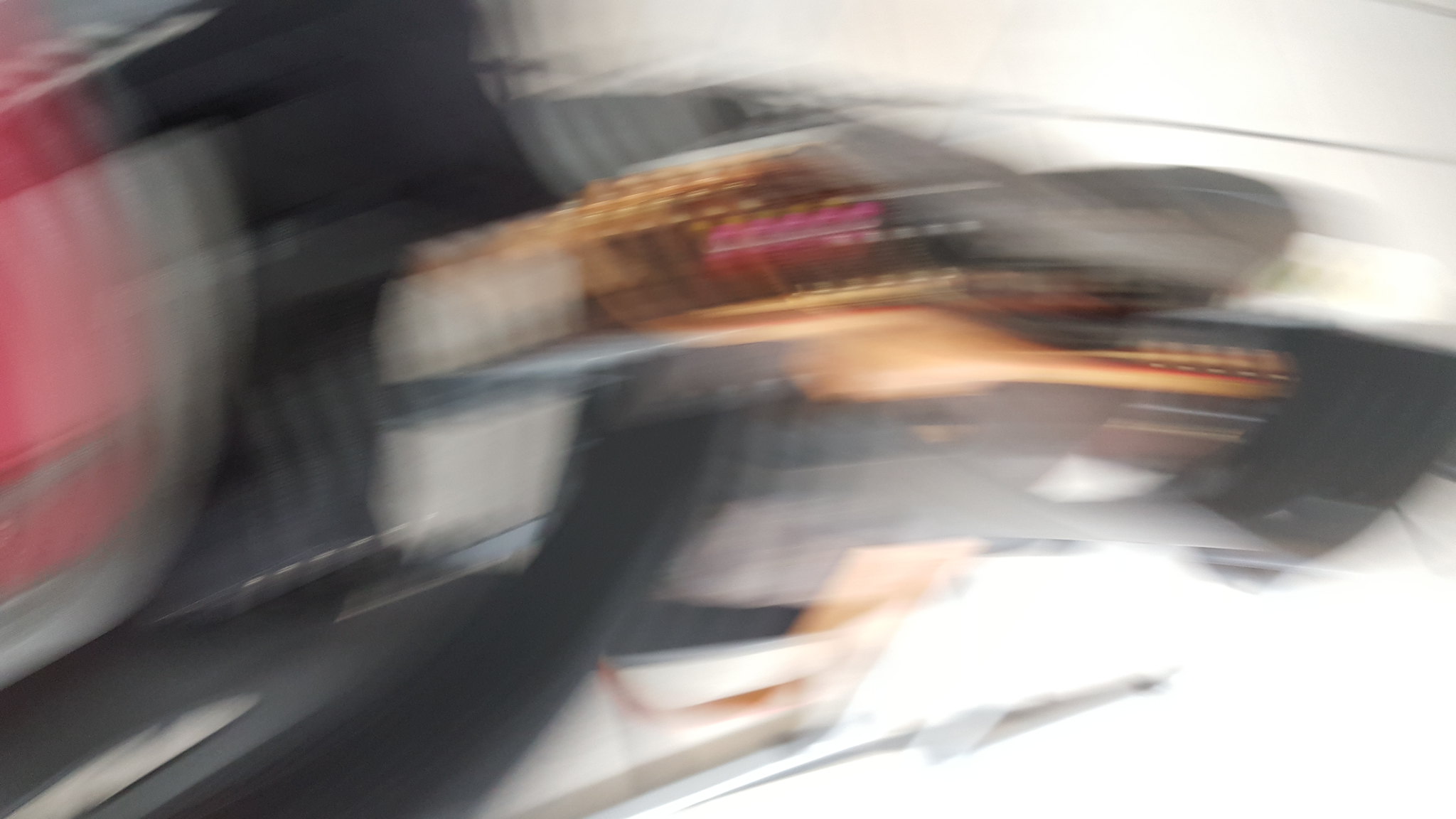This image is a very blurry, horizontally-oriented photograph, characterized by significant movement, likely taken while in motion. The scene is difficult to discern due to its out-of-focus nature; however, a few details emerge. There appears to be a black container or perhaps a vehicle with red accents, possibly a taillight, set against a white background. There is also a suggestion of a brown bag resting atop this container or vehicle. Moreover, some viewers mention a reflection that might indicate the underside of a chair or a car mirror image. The colors present in the image include black, red, white, brown, orange, and pink, with hints of sunlight or a light blue sky in the backdrop. A possible car is noted, with some describing a man in a red shirt and black pants, suggesting he might be wiping or polishing the car. However, exact identification remains elusive due to the extreme blurriness and motion captured in the photo.